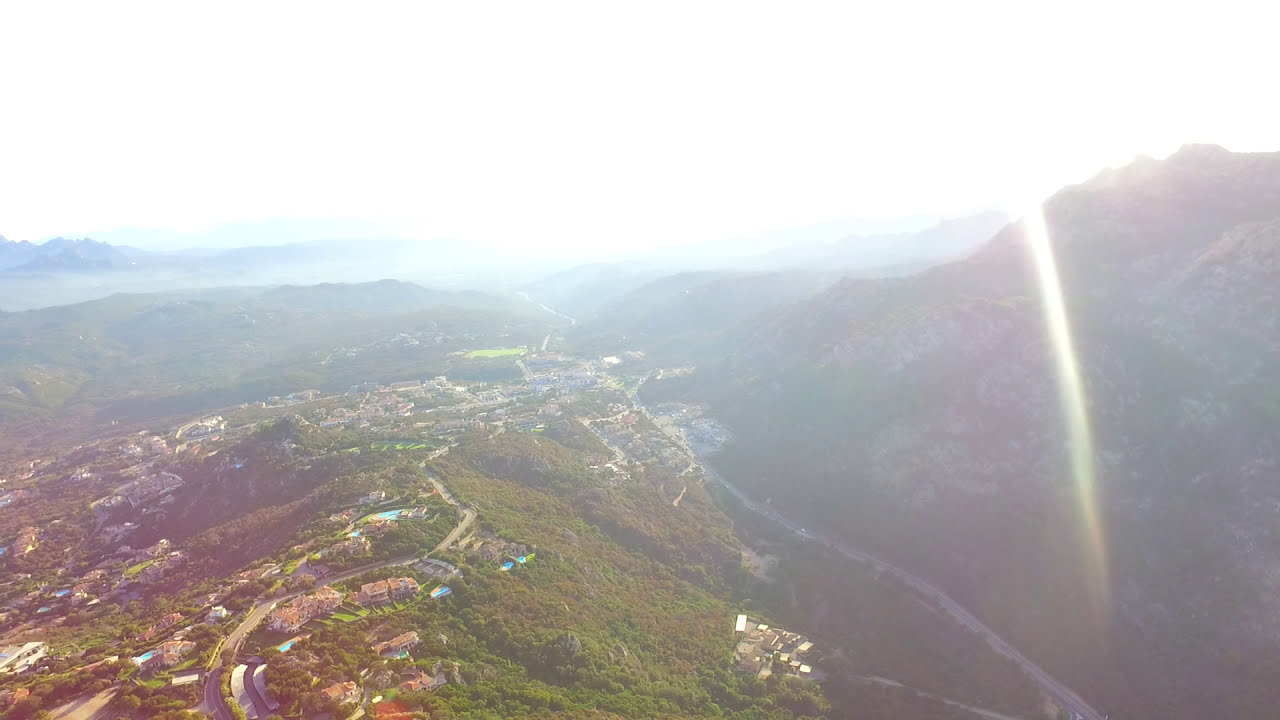The image captures an expansive aerial view of a lush, mountainous valley with a vibrant rainbow arching over the scene. The image is very wide and rectangular, featuring a predominantly white sky at the top transitioning into a light gray and blue horizon, which hints at a distant mountain range. On the right side, a large green and brown hill is prominent, with a winding road that extends from the hill and disappears into the bottom right corner. This road divides the landscape, which is dotted with numerous homes, many featuring swimming pools filled with light blue water, indicating a possibly affluent residential area.

The valley itself, situated towards the bottom right, is traversed by multiple roadways converging from the bottom left and right corners of the image. The landscape is a patchwork of green and brown spaces interspersed with trees and additional road networks that weave through the valley, extending toward the built-up central area in the distance.

The mountain on the right side casts a shadow, as the sun shines brightly behind it from the top right corner, sending rays of light through the valley. The backdrop is filled with the soft outlines of additional hills, mountains, and valleys, creating a picturesque scene. The partially visible rainbow begins near the bottom right, adding a touch of vibrant color to the serene and expansive scenery.